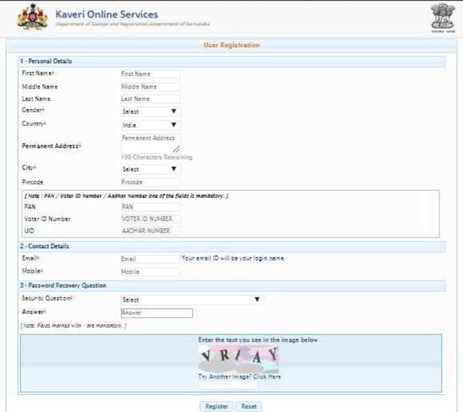The image is a grainy screenshot of a registration interface for an application named "Kavari Online Services." The form is titled "User Registration" and is divided into several sections for collecting user information.

The first section, "Personal Details," includes text boxes for entering:
- First Name
- Middle Name
- Last Name
- Gender
- Country
- Permanent Address
- City
- One additional field, possibly a postal or zip code

Following this, a line of text is almost completely unreadable. The readable entries that follow include text boxes for:
- PAN (Permanent Account Number)
- Visitor ID Number
- UO (Possibly another form of identification number)

The second section, labeled "Contact Details," prompts the user to provide:
- Email Address
- Mobile Number

The third section, "Planned Recovery Question," contains a secure question feature. A drop-down menu allows users to select a security question, and a text box allows them to type in their answer.

At the bottom of the form, users are instructed to "Enter the code in the image you see below." The code displayed is "VRIAI."

Finally, two buttons are available at the bottom center of the page for form submission:
- Register
- Reset